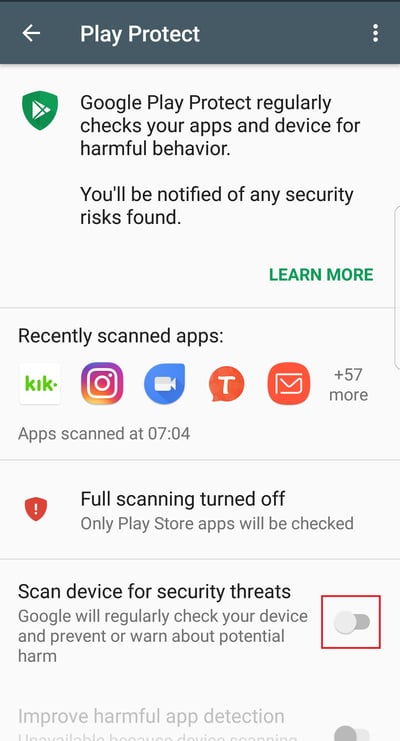The image is a screenshot from a mobile phone, oriented in portrait mode with a height approximately 2.5 times its width, resembling the proportions of a standard cell phone screen.

At the top, there is a horizontal blackish-gray bar with white text. On the left side of this bar, there is a back arrow icon. In the center, it reads "Play Protect," and on the right, three vertical dots indicate a menu for additional options.

Below this bar, a horizontally bordered section features a green shield icon with a play button in the center. Accompanying the icon is a message in black text: "Google Play Protect regularly checks your apps and device for harmful behavior. You'll be notified of any security risks found." At the bottom of this message, green text reads "Learn More."

Following this section, there is a list of recently scanned apps, which includes Kik, Instagram, Reels, Temu, and Google Mail, alongside a note that indicates there are "plus 57 more" apps scanned. A timestamp shows that these apps were scanned at 7:04.

Below the scanned apps list, a red shield icon with a white exclamation mark alerts users, stating "Full scanning turned off." Underneath this alert, there is a boxed section with the text "Scan device for security threats," accompanied by a toggle switch that is in the 'off' position and highlighted in red.